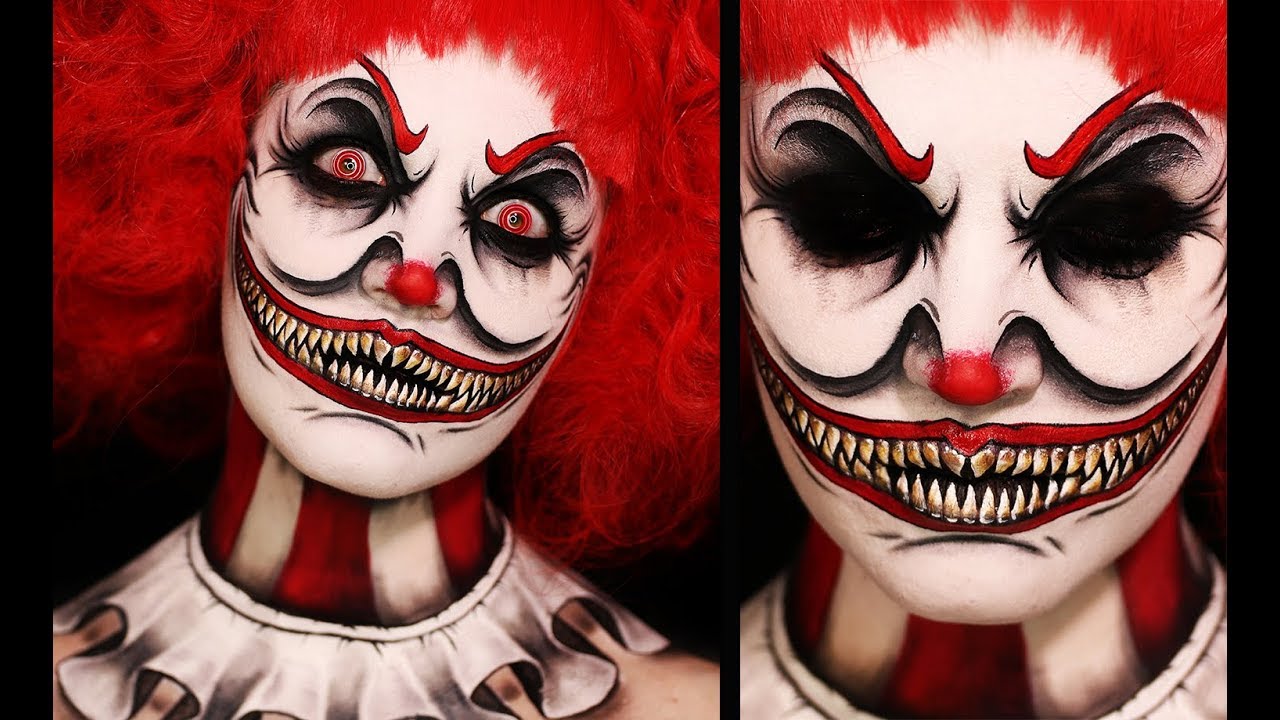This AI-generated, photorealistic image portrays an exceptionally terrifying clown divided into two sections. On the left, the sinister clown stares directly ahead, its menacing gaze accentuated by red eyes framed with exaggerated red eyebrows atop thick black makeup. The clown's large, frizzy red hair encircles its face, crowned by a prominent red nose. Its gruesome mouth stretches unnaturally wide, nearly reaching the ears, revealing sharp, rotting teeth set against a black backdrop. The neck is adorned with a black and white pattern and topped with a white ruffled collar. On the right, a closer and even more horrifying depiction reveals the same clown with its eyes now gaping, empty black holes, intensifying its evil presence. This vivid imagery, featuring the red hair and distorted facial features, starkly illustrates a nightmarish, horror-themed clown.